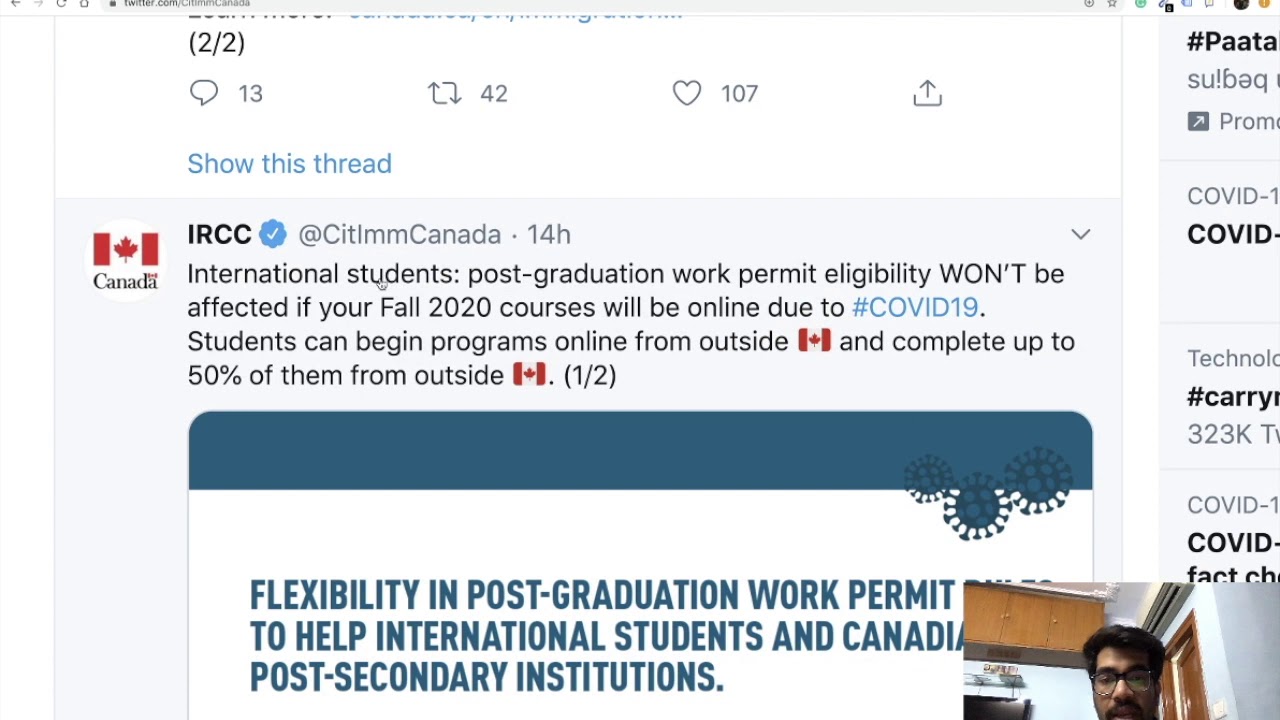A screenshot from Twitter is partially visible, with the top section cut off. In the top left corner, there's a white horizontal rectangular box displaying "2/2." Below it, the number 13 appears next to a reply icon. Further right, the number 42 is shown. Moving further right, there is a favorite (heart) icon with the number 107 beneath it. At the far right, there's an upward-facing arrow with a half-box underneath for forwarding the thread.

In the main portion, on the left side, there is a circular icon containing the Canadian flag, with the word "Canada" below it. To the right of this icon, a post is presented by "IRCC" in capital, bold black letters, followed by "@CitImmCanada," posted 14 hours ago. The post reads: "International students, post-graduation work permit eligibility won’t be affected if your Fall 2020 courses will be online due to #COVID19. Students can begin programs online from outside " (with a Canadian map icon representing the word "Canada") "and complete up to 50% of them outside of" (another Canadian map icon).

Below this, a small rectangular box features a blue top section, while the remainder is two-thirds visible with the bottom cut off. Inside, a blue bold header reads "Flexibility in Post-Graduation Work Permit." The text below mentions provisions to help international students and Canadian post-secondary institutions, though some words are cut off.

To the right of this text box, an image of a person with olive skin, dark hair, glasses, and a dark mustache is displayed.